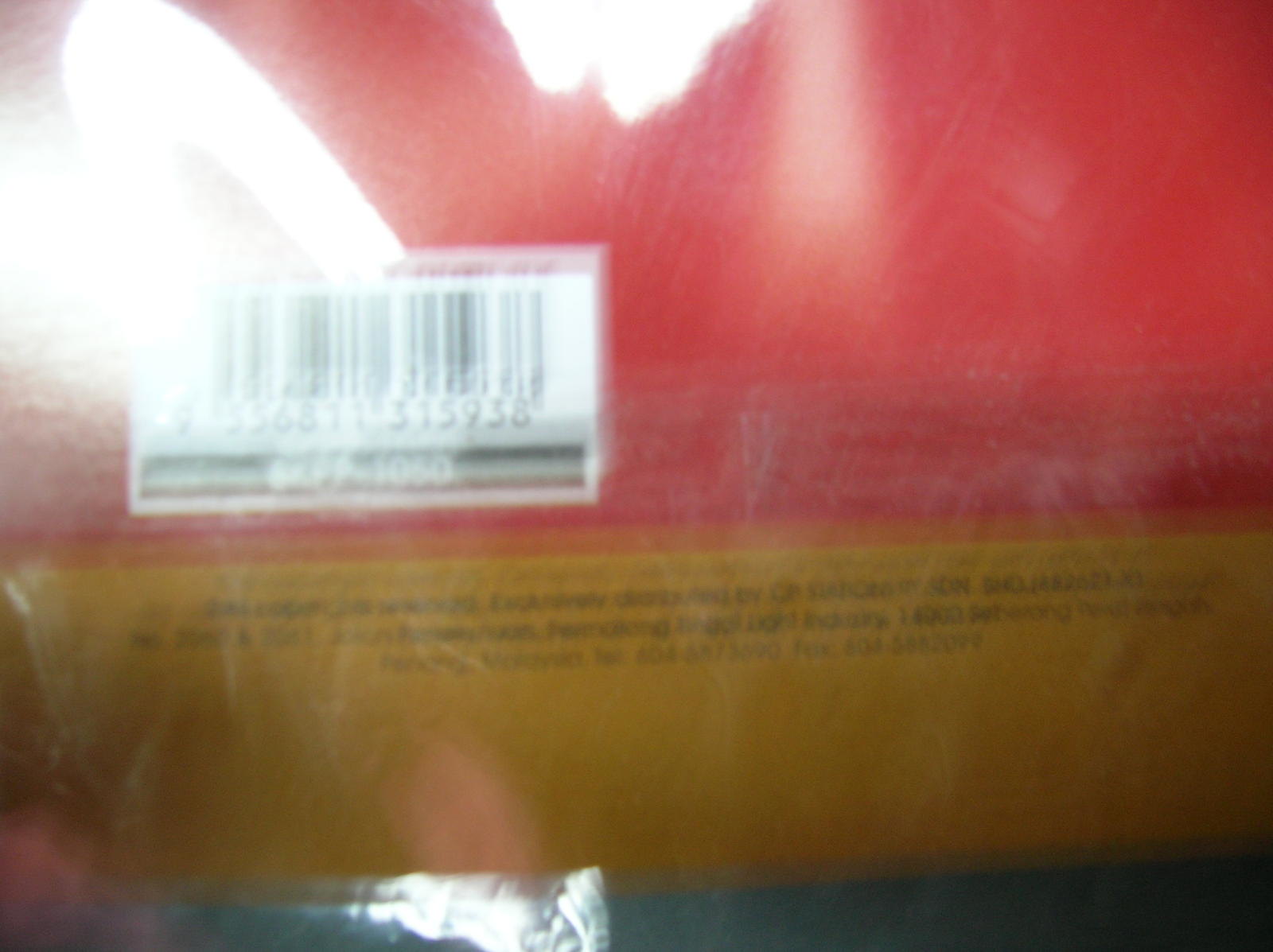The image depicts a box with a blurred focus, centering predominantly on a UPC code. The box features a distinct color scheme; the upper part is red, curving downwards to a yellow bottom. This red area of the box also catches light reflections, notably a bright spot at the upper center and additional reflections towards the left side. The yellow section contains some writing, although it is indiscernible due to the blurriness. The UPC code, meant to be the focal point, is situated on the left side of the red upper section of the box.